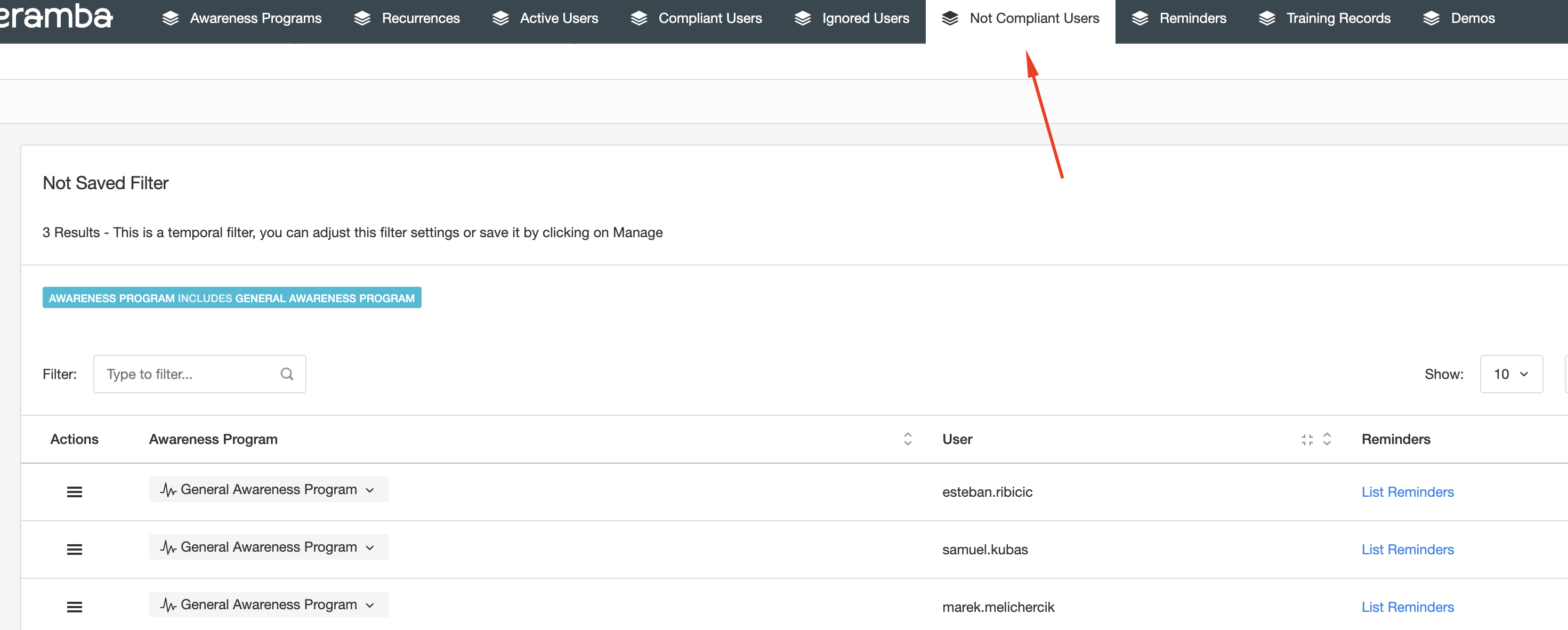Here we have a screenshot of a webpage related to user compliance and awareness programs. The left edge of the screenshot is partially cut off, making it difficult to discern the exact title; it might be something like "E-Ramba," but some letters are missing and it's unclear. 

The webpage features a black banner at the top with a distinctive font used for the letters "A." The banner includes various menu options: "Awareness Programs," "Recurrences," "Active Users," "Compliant Users," "Ignored Users," and "Noncompliant Users," the latter of which is currently selected and indicated by a red arrow. Additional options include "Reminders," "Training Records," and "Demos."

Below the banner, the highlighted "Noncompliant Users" section shows a warning about a "Not Saved Filter" with three results displayed. The filter is described as temporal, allowing users to adjust settings or save the filter by clicking on "Manage." 

Further down, a blue rectangle provides details under the "Awareness Program" header, including a sub-section for "General Awareness Program" with an associated filter showing "10+" results, though only the top three are visible. The visible entries all pertain to "General Awareness Programs" and list three different users.

Overall, the screenshot seems to be part of a management or oversight tool focusing on user compliance within various awareness programs.